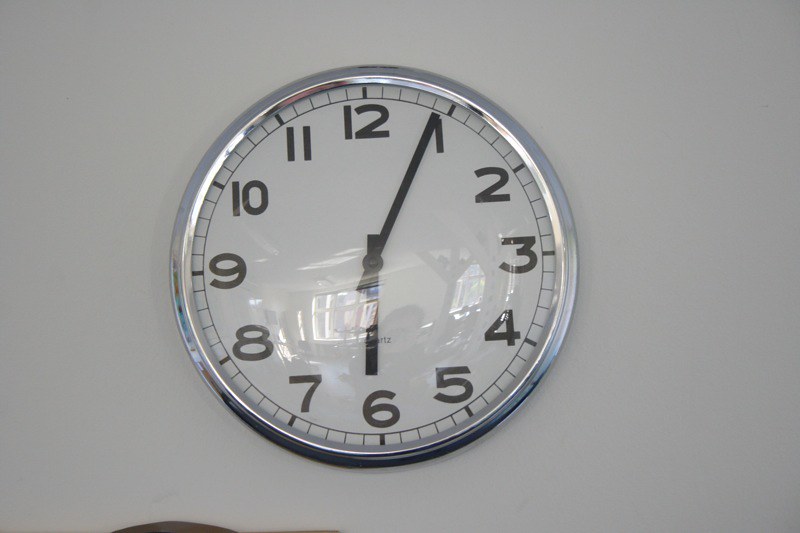This image displays a minimalist scene featuring a sleek, chrome-finished clock mounted centrally on a pristine white wall. The clock's face is also white, presenting a striking contrast with its black numerals, which span from 1 through 12. At the current time, the hour hand is precisely at 6, while the minute hand is positioned between the 4 and 5, indicating that it is approximately 6:22. Surrounding the numerals, a series of black markers further accents the design. Each hour is denoted by a prominent dark bar, and intervening minutes are marked by lighter bars, with slightly darker bars at 5-minute intervals for added clarity. The overall composition exudes a modern and orderly aesthetic.